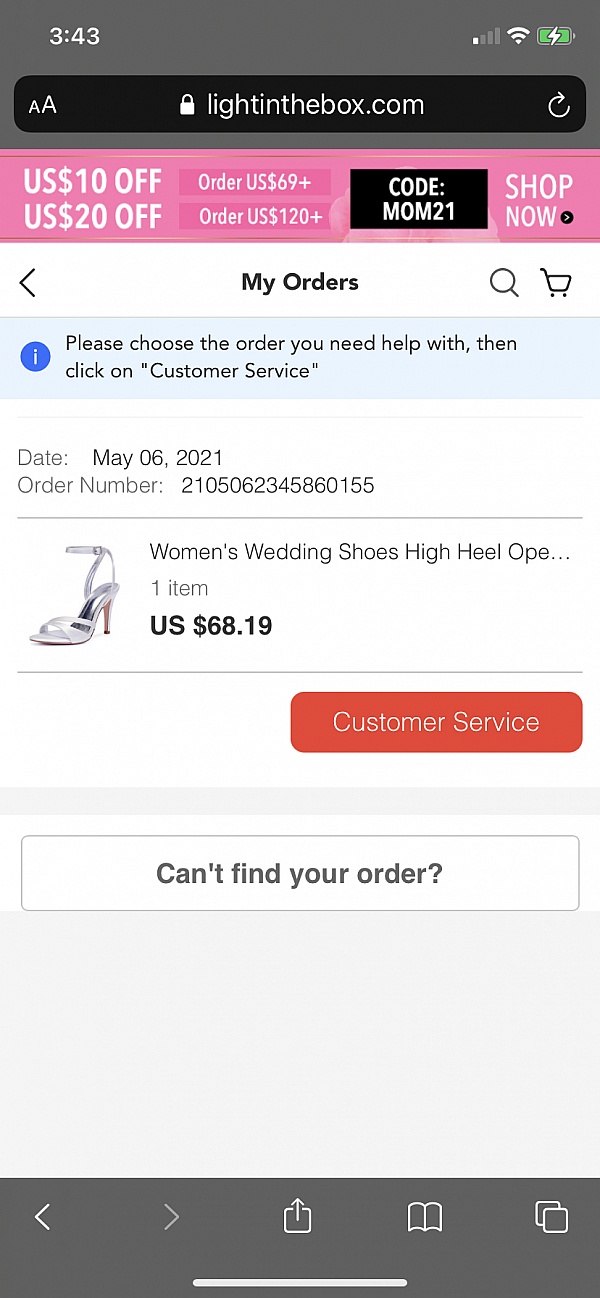Screenshot of a smartphone displaying a webpage from LightInTheBox.com. The smartphone interface shows a green background with white text at the top left corner reading "343", alongside icons indicating a single cell signal, full WiFi, and a charging battery in green.

Below this, there is a darker green address bar featuring two "A" icons on the left (one uppercase and one lowercase), a padlock icon in the center, and the website URL "lightinthebox.com". To the right of the address bar is a refresh icon.

An advertisement banner follows, presented in a white and pink color scheme, with text offering discounts: "US $10 off, US $20 off on orders $69+, US $120 off". A black box with the code "MON21" in white text is also present, alongside a "shop now" call to action in white text on a purple-pink background.

Navigational elements are present on the page, including an arrow pointing left labeled "my orders", a magnifying glass icon (search), and a shopping cart icon. Below this, black text on a white background instructs users to "please choose the order you need help with and click on customer service".

Next, there is an order section with specific details: the order date "May 6th, 2021", and an associated order number (not displayed). The order includes a pair of gray or silver high heels labeled "women's wedding shoes, high heel O...", priced at "US $68.19". A red button labeled "customer service" with white text is visible at the bottom right, next to a message stating "can't find your order".

Finally, the screenshot includes the browser's bottom navigation bar with icons for back, forward, refresh, bookmarks, and tab view.